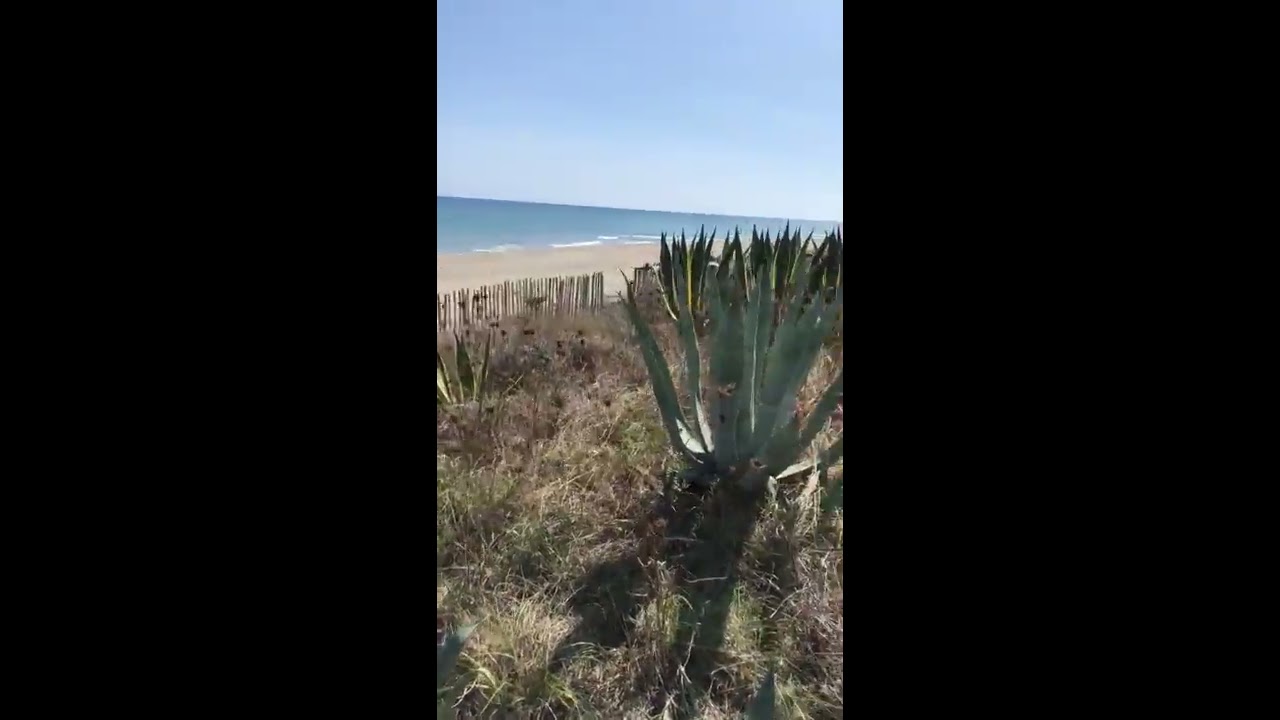The image captures a serene beach scene viewed from an elevated vantage point. In the foreground, a striking desert plant with straight, pale green leaves edged in a deeper green commands attention, casting a shadow on the ground. This plant, which resembles a cactus or an agave, is surrounded by sparse, dead grass and other spiky, cactus-like shrubbery. A stick-like, wooded fence can also be seen near the plant. The background reveals fine sand with gentle, white-capped waves lapping at the shore, progressing into clear, light blue ocean waters. The horizon is defined by the meeting of the ocean and the sky, which occupies the top third of the image. The sky is a vibrant blue, devoid of clouds, hinting at a sunny, daytime setting. Thick black rectangles border the left and right sides of the image, framing the central focus.